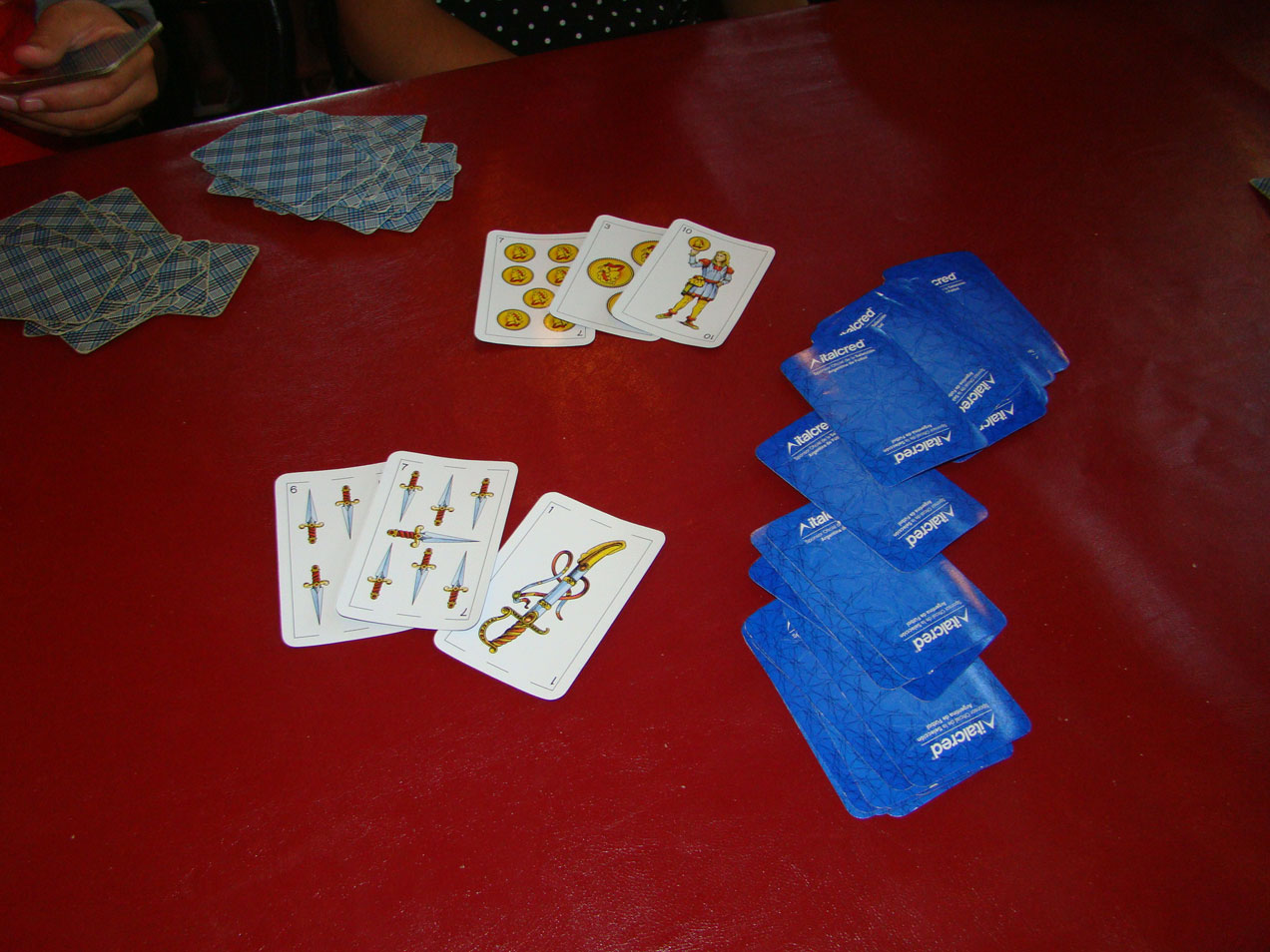A detailed layout of a dark brown table covered with playing cards. In the center of the table, a set of six unique playing cards is arranged in two rows of three. The top row features cards adorned with medieval figures and gold coin-like objects, while the bottom row displays cards with images of small swords and knives. To the top left of the image, two stacks of cards are placed face-down, revealing a light blue and white checkered flannel pattern on their backs. On the right side of the table, another stack of playing cards lies face-down, displaying dark blue backs. In the top left corner of the photograph, two people are partially visible; one individual holds a cell phone, and next to them, a person wearing a black and white polka-dotted top is seen.